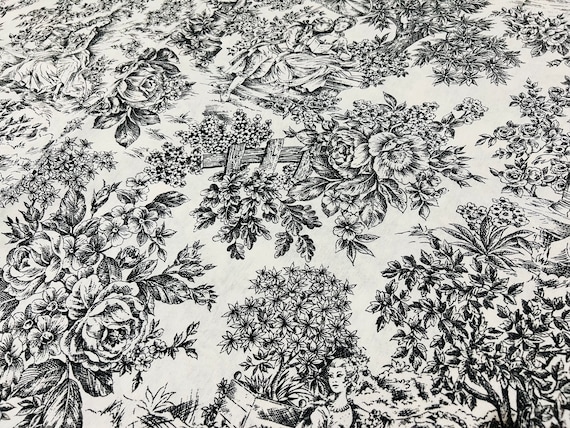The image features a detailed black and white floral print, resembling an intricate ink drawing on paper. The design is densely populated with large blossoms, leaves, and various plants creating a rich, botanical tapestry. Dominating the lower portion of the image, there's a silhouette of a woman dressed in 1800s attire with short hair, adorned with a white and black necklace. Nearby her is a box or pot overflowing with flowers, which includes a tree growing out of it. This woman’s head appears small in comparison to the massive flowers surrounding her. Positioned towards the upper part of the image, a young couple is depicted. The woman, dressed in a white blouse, appears to be seated on a chair or bench, reading a book, while a man, possibly an English gentleman, leans against her shoulder. This upper group is also ensconced in the floral scenery. The entire composition is monochromatic, emphasizing the shapes and lines of the abundant botanical elements.